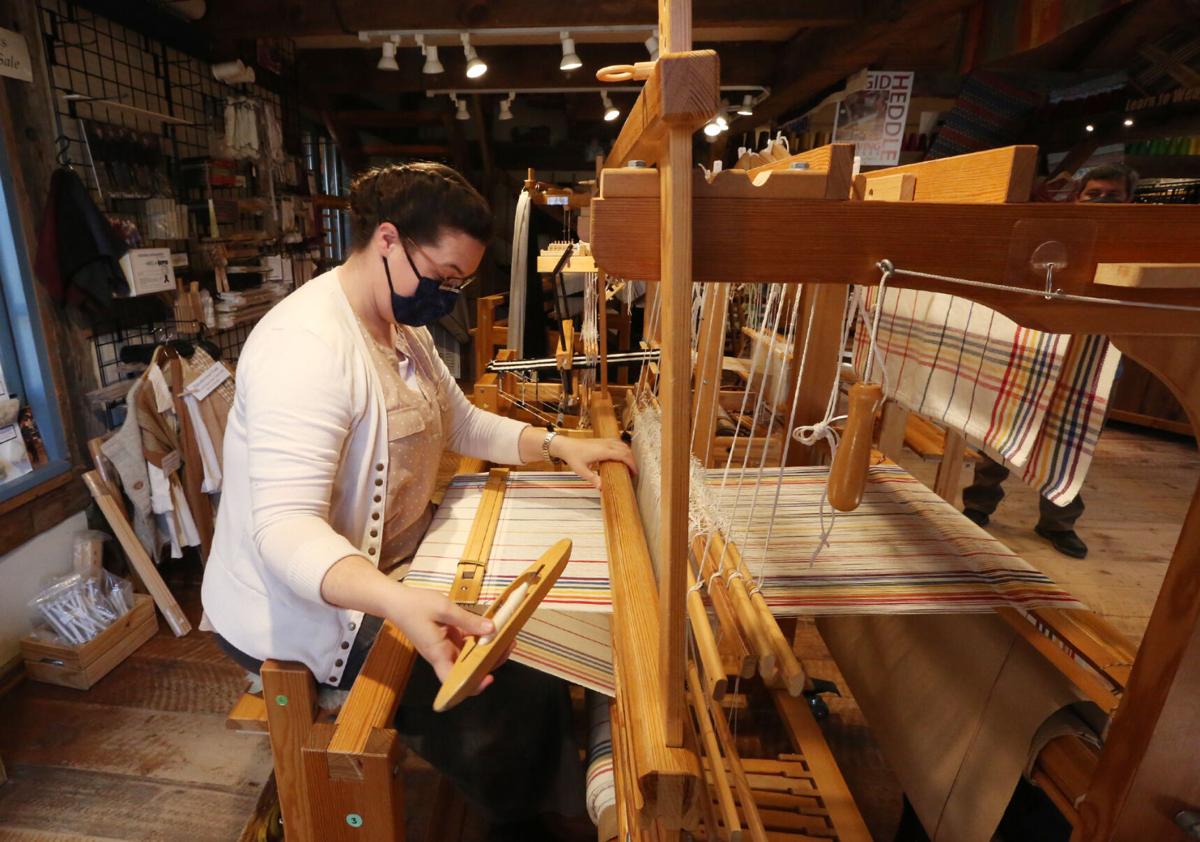The color photograph, in landscape orientation, captures a detailed moment inside a well-lit, rustic workshop with well-worn wooden floors. The main subject, a woman with light skin and brown hair pulled back into a French braid with a bun, stands to the left side, intently focused on her work at a large wooden loom situated to the right side of the image. She's wearing glasses, a black face mask for either fiber protection or disease prevention, a cream-colored blouse under an unbuttoned white cardigan. The fabric she is weaving is predominantly white, interwoven with red, yellow, green, blue, and purple crisscrossing stripes, and appears to be quite wide, supported by the expansive loom. In her right hand, she holds a wooden shuttle with a spool of thread. The room is well-organized with materials stacked against the walls and on shelves, illuminated by ceiling track lighting. Bright natural light streams in through a couple of visible windows, enhancing the intricate details and creating a vibrant atmosphere.